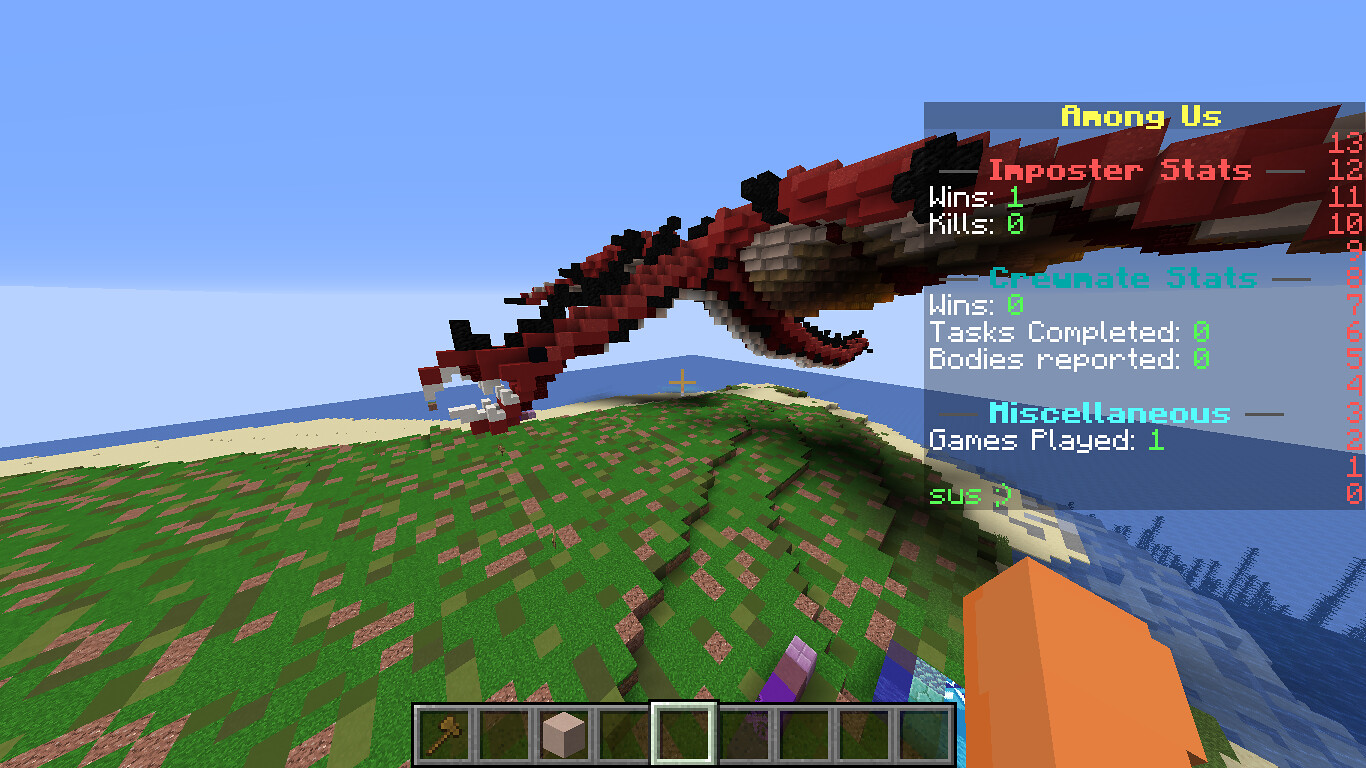The image is a screenshot from the game Minecraft, featuring a distinct pixelated animation style with characteristic blocky graphics. It portrays a landscape with green grass studded with pink square flowers and a large body of blue water. The sky is mostly light blue, transitioning to darker hues towards the top of the screen, indicating a sunny day. Central to the image is a red, burgundy-colored dragon-like creature with its mouth open. To the right, there's an orange building, and in the grass, a religious cross is evident.

At the top of the screen, a blue box displays the text "Among Us" in yellow, followed by "Impostor Stats." Below, the stats include "Wins: 1, Kills: 0," and additional game statistics such as "Tasks Completed: 0" and "Bodies Reported: 0." The term "SUS" also appears among other numbers and details. At the bottom of the screen, the player’s equipment is visible, including icons for an axe and a block among nine inventory slots.